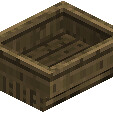The image displays a pixelated, wooden box-like object reminiscent of items found in the game Minecraft. The box is viewed from an angled, top-down perspective, allowing a glimpse inside. The interior of the box appears to be constructed from small wooden boards. The rim of the box is a lighter brown, while the interior and base are a darker shade of brown. The pixelated texture is evident across the entire box, emphasizing its video game aesthetic. The sides of the box seem to be slightly cropped, indicating the object is not fully within the frame. The box is set against a plain white background, providing contrast and highlighting its pixelated design.